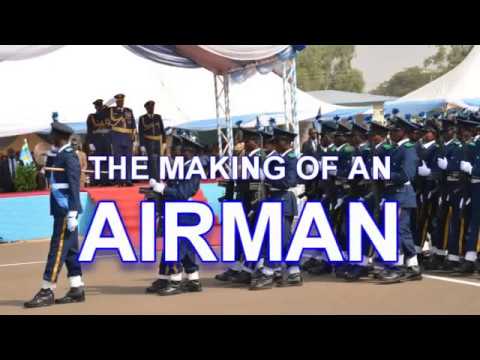The horizontally aligned, rectangular image features a military scene bordered by black strips at the top and bottom. The central focus is a group of soldiers in dress uniforms, marching in formation from right to left on a gray street marked by white lines. The soldiers wear navy blue jackets and pants with gold stripes down the legs, complemented by white gloves and either white socks or cuffs. Their blue hats are topped with plumes.

In the foreground, a leading soldier faces left, guiding the formation which spans multiple ranks. A text overlay in all caps reads "THE MAKING OF AN AIRMAN," with "AIRMAN" in larger, white text outlined in bright blue.

In the background, there’s an elevated viewing stand with a red-carpeted stairway, where three highly decorated officers stand under a canopy. One officer salutes, while the others stand at attention. The event appears to be a celebration or graduation, with additional tents and canopies visible, suggesting a formal occasion. Notably, all participants in the scene—the marching soldiers and the saluting officers—are Black men, adding a layer of cultural significance to the military display.